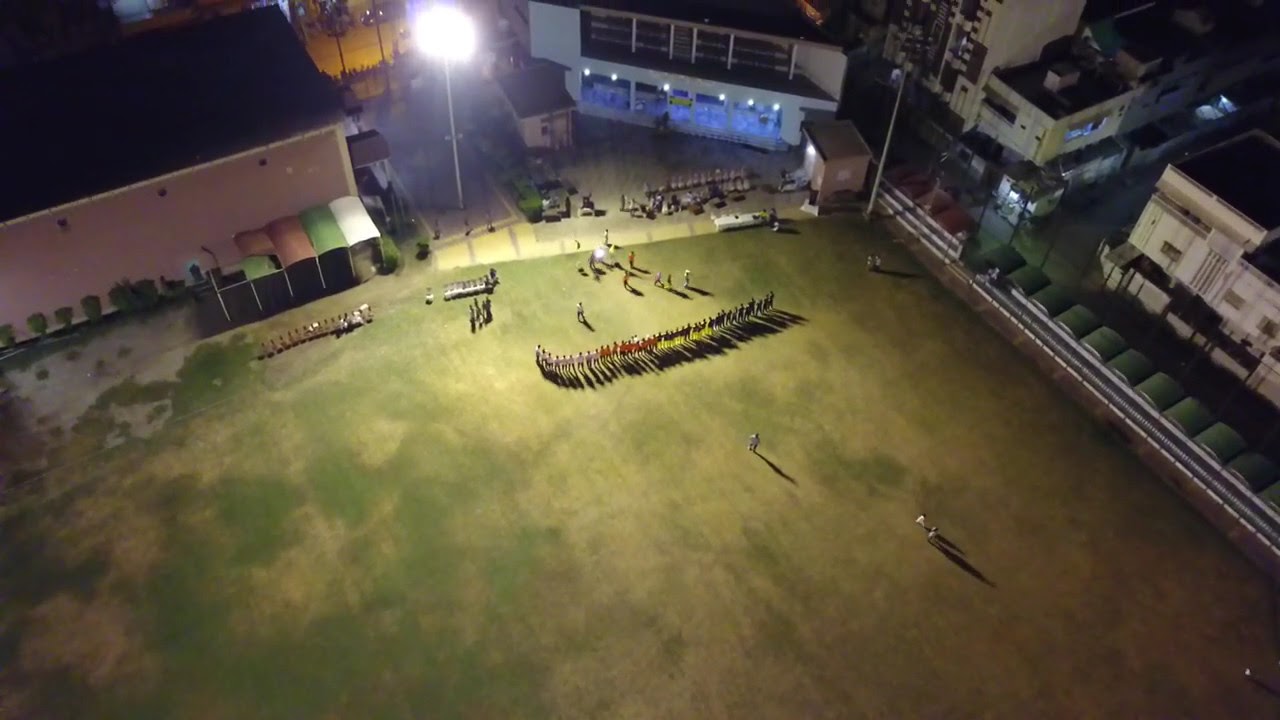An aerial nighttime view reveals a well-lit green playing field bordered by tall buildings, possibly a school or apartments. In the upper middle section of the image, a line of roughly fifty people, likely players in uniforms, stands facing the top of the image. The uniforms vary: some wear darker clothes, others have bright green pants with red shirts, and another group is dressed in white. A tall pole in the center casts a bright light, creating shadows of the standing figures on the field. Portable toilets with green rooftops are visible on the right edge, hinting at a recent or upcoming event, while yellow and blue lighting from nearby structures adds depth to the scene. The organized line and the presence of uniforms suggest a sports practice or gathering, with no active game in progress.